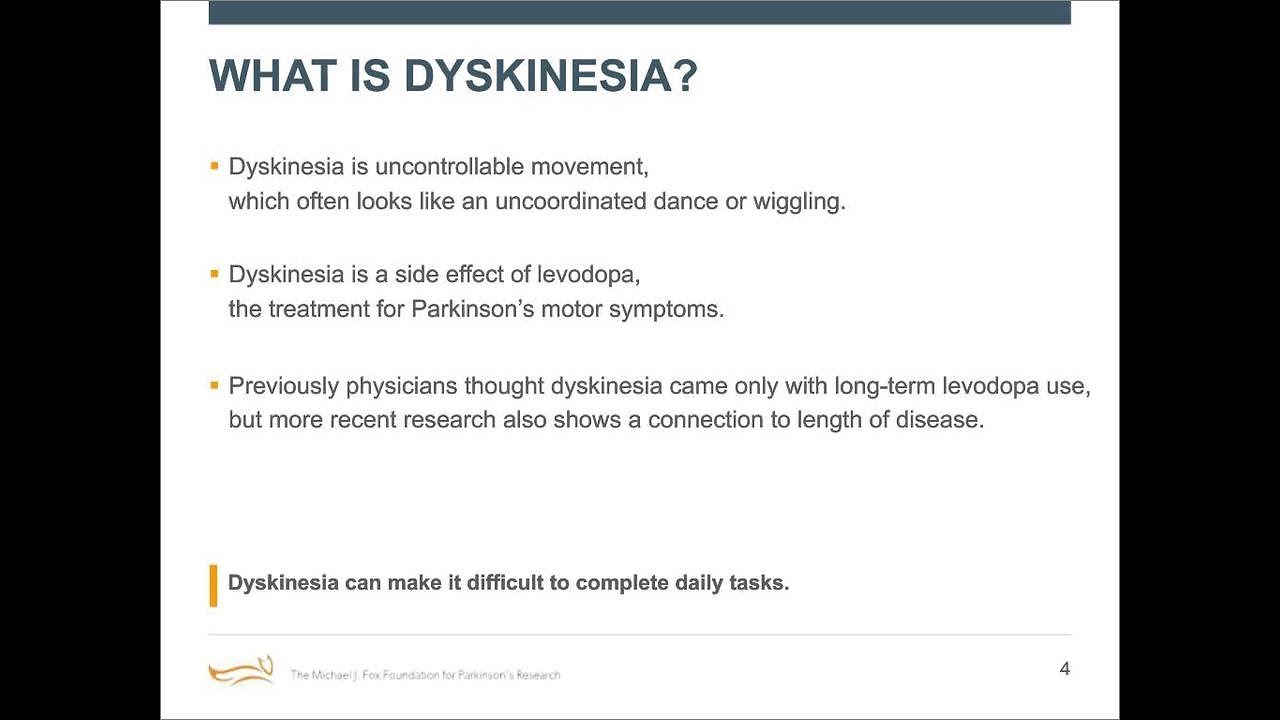A screenshot from an educational material by The Michael J. Fox Foundation for Parkinson's Research, framed with thick black vertical borders on both sides. At the center is a white page with a dark blue header, which contains the title "What is dyskinesia?" written in bold, all-capital letters. Below the header, there are three bullet points, each marked by small orange dots. The text is in a regular blue font and explains the following:

1. Dyskinesia is an uncontrollable movement, often resembling an uncoordinated dance or wiggling.
2. It is a side effect of levodopa, a treatment for Parkinson's motor symptoms.
3. Although it was previously believed that dyskinesia occurred only with long-term levodopa use, more recent research indicates it is also connected to the length of the disease.

There is a notable amount of blank space following the descriptive text. Adjacent to a vertical orange bar, in bold text, it reads, "Dyskinesia can make it difficult to complete daily tasks." A thin, faint horizontal line separates this statement from a logo at the bottom of the page. The logo, featuring an outline of a fox, confirms it is indeed from The Michael J. Fox Foundation for Parkinson's Research. The number "4" appears on the right-hand side, suggesting this is page four of the educational document.